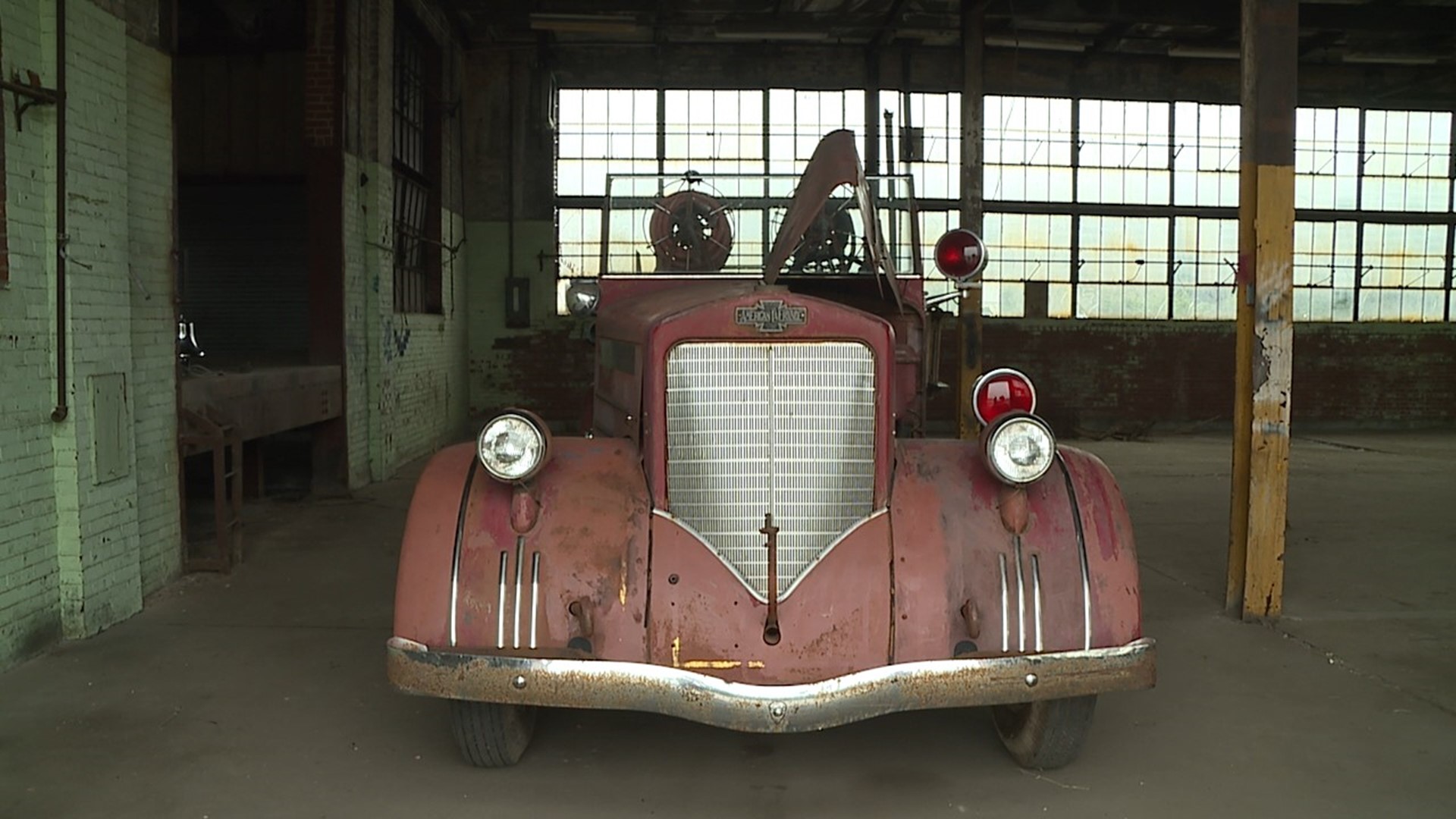The image shows a vintage firetruck, parked inside a garage or warehouse. The background features rows of factory-like windows, with a white brick wall on the left and a yellow steel beam on the right. The firetruck itself is a faded, dull red with patches of rust, suggesting it needs restoration. Prominently, it has a chrome bumper with visible wear below a silver grille, which features an emblem above it. The front is marked by two headlights that stick up slightly; behind the right headlight is a red light, with another swivelling red light next to the driver's door. There's also a discernible hand pump with a metal handle at the back. The overall color palette consists of grays and browns from the surroundings, contrasting with the faded red and silver of the firetruck.